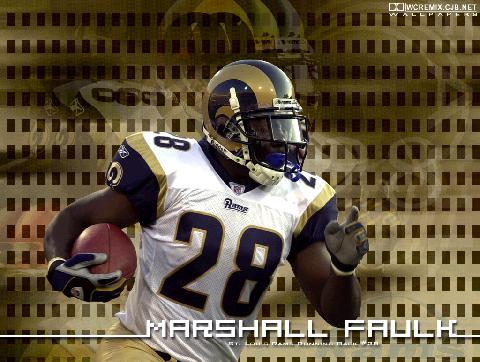This detailed computer wallpaper features legendary St. Louis Rams running back, Marshall Faulk, sporting his iconic number 28 jersey. The white jersey is accentuated by blue and gold shoulder pad detailing, including a ram’s head emblem with curling horns. Faulk, an African American athlete, is seen cradling a brown football in his right arm and wears black and gray gloves. He’s captured in mid-action, looking to his left with the background featuring a larger, layered image of him. The backdrop also includes a pattern of golden squares resembling scantron sheets, interspersed with darker gold brick designs. His name, "Marshall Faulk", is written in a white, pixelated, tech-style font from that period, prominently displayed along with the text "w cremix cbj.net. wallpaper" at the top right corner.